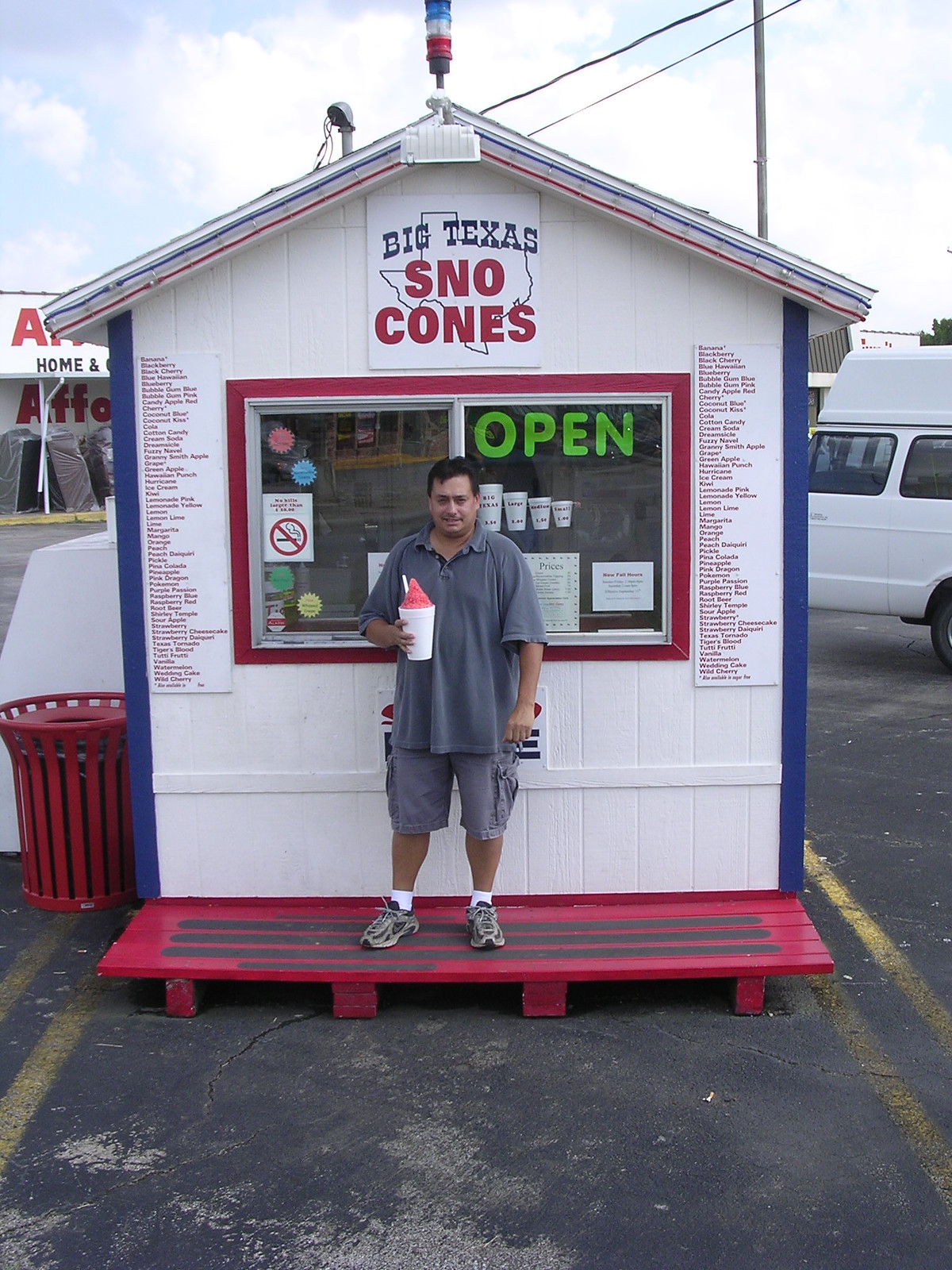In this detailed image, a man is posing in front of a quaint, makeshift snow cone booth that appears to be set up in a blacktop parking lot, evidenced by the yellow parking stripes on either side. The booth resembles a small white house-like structure, with subtle blue stripes on its walls and a uniquely curved triangular roof adorned with blue and red stripes. Above a prominent large central window framed in red, a sign proclaims "Big Texas Snow Cones" in bold letters, accompanied by the outline of Texas. Flanking the window are two columns listing various menu items available for purchase. Additionally, signs indicating the booth's open status, no smoking rules, and cup sizes are visible on the window. 

The man, dressed in a gray polo shirt and gray cargo shorts, stands on a red platform detailed with black stripes, evocative of pallet boards used for stairs. He's wearing white ankle socks and grayish-black shoes, and he sports black hair. In his hand, he holds a large red snow cone, presented in a white styrofoam cup with a straw poking out, the vibrant colors of the snow cone contrasting sharply with his attire and the booth behind him.